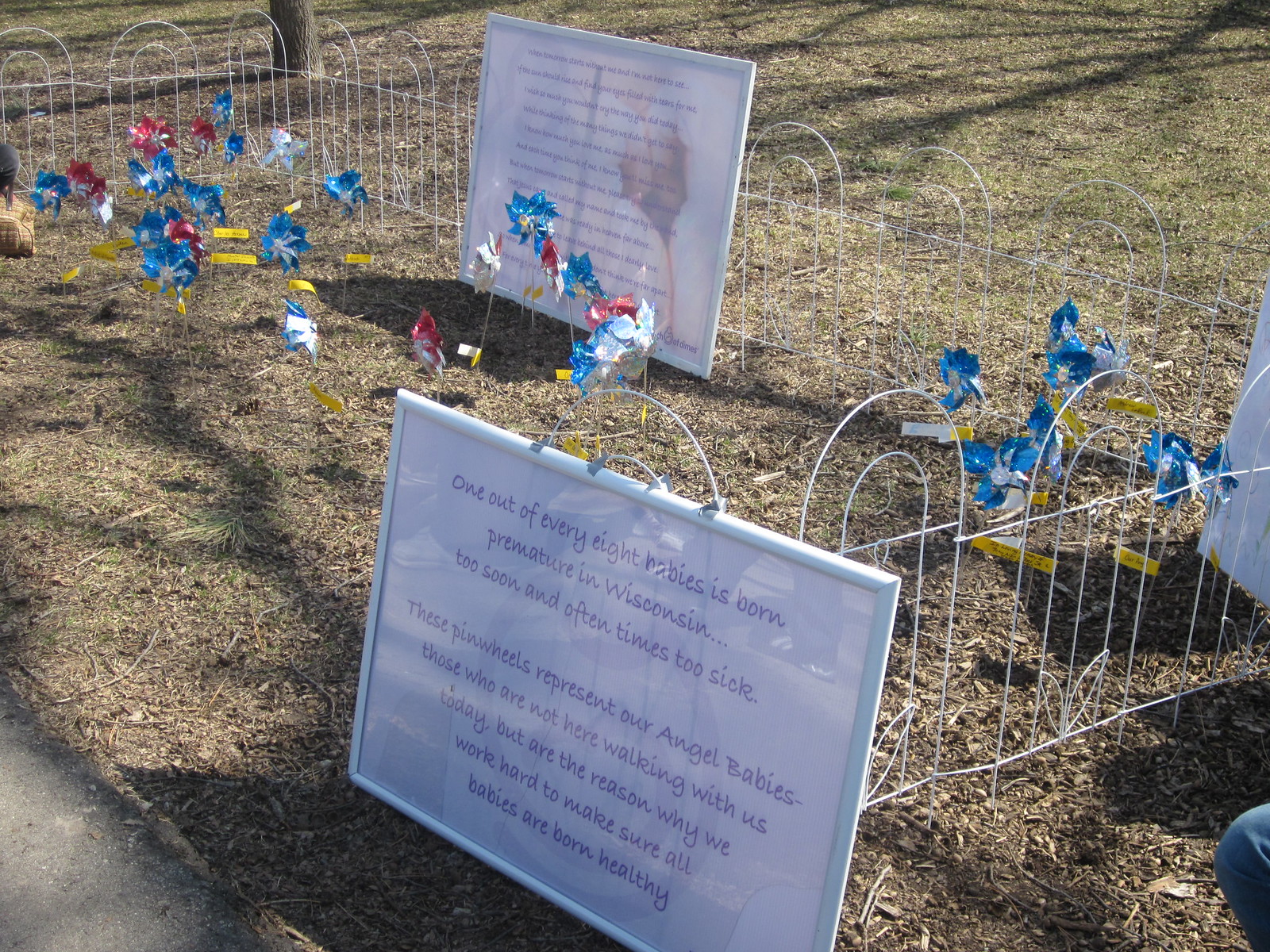The image captures a memorial display set in an outdoor environment with brown, dead-looking grass, suggesting a fall or early winter setting. The focal point is a small section of land fenced in with low, rounded, white wire panels, roughly a foot to two feet tall, often used to section off garden areas. Inside the fenced area, vibrant pinwheels in blue, red, pink, and white, each affixed with yellow tags possibly bearing names, stand in striking contrast to the muted grass. These pinwheels are described as shiny and sparkly. Prominently displayed is a large white sign with a white frame and light blue text that reads: "One out of every eight babies is born premature in Wisconsin, too soon and oftentimes too sick. These pinwheels represent our angel babies, those who are not here walking with us today, but are the reason why we work hard to make sure all babies are born healthy." Another similar sign is visible but partially obscured in the background. The scene is anchored by a single tree, adding to the somber but poignant atmosphere of the memorial.